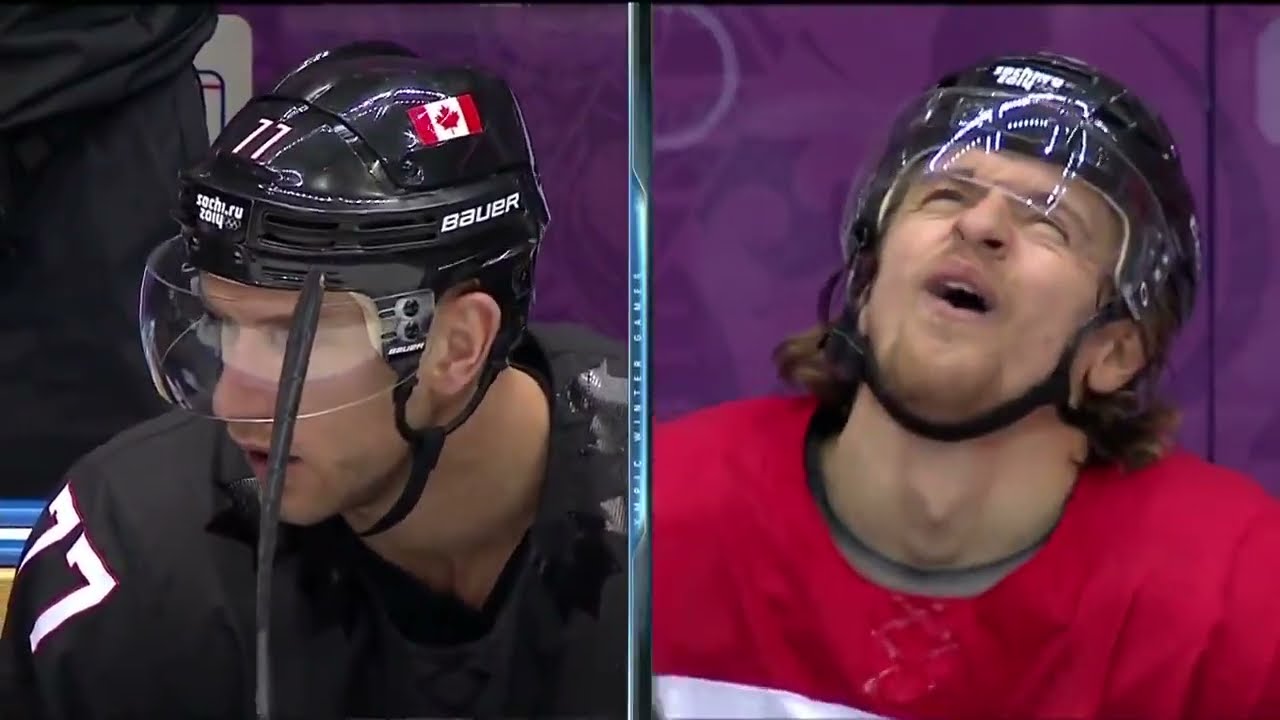The image depicts two hockey players in a horizontally rectangular frame, split by a vertical line into two sections. The background is predominantly purple with white and blue lines, and there are hints of yellow in the left section. The player on the right is wearing a red and white jersey with a black helmet and a black chin strap. He has a little chin beard and long brown hair that flows out from under his helmet. He is looking upward with his mouth open, suggesting either surprise or pain. The player on the left is dressed in a black and white jersey, bearing the number 77, and his helmet is also black with a clear visor. The brand name BAUER is visible on the helmets. This player lacks facial hair and appears to be glancing towards the left side of the image. Both players are captured in a moment that seems to be a reaction to an event off-camera, possibly during a sporting event broadcast.